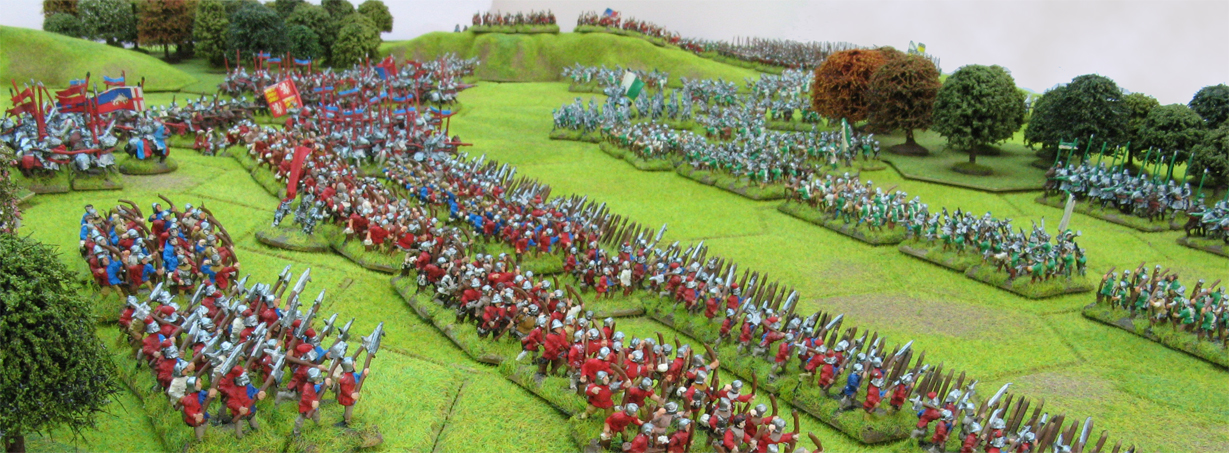The image is a horizontally aligned rectangular depiction of a battlefield model, featuring detailed toy soldiers and lush greenery. On the left side, three distinct rows of soldiers in red uniforms and silver helmets brandish silver swords. To the right, a front row of soldiers in green and silver uniforms faces them, with an additional row partially visible behind. Both sides are embellished with perfectly round tree branches anchored to green bases, positioned on the upper right, upper left, and partially on the lower left of the image. The battlefield itself is a zigzag pattern of green grass, adding a naturalistic touch. Further back, atop a hill, more soldiers clad in red uniforms are seen, framing the scene against an overcast gray sky. The juxtaposition of the well-maintained landscape and the poised toy soldiers creates a vivid and dynamic representation of a historical battle moment.